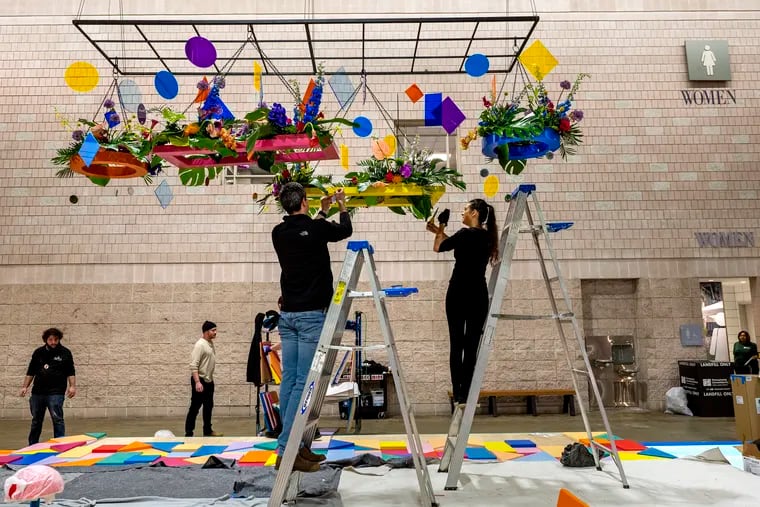The image depicts a bustling scene inside what appears to be a gymnasium with beige brick walls. At the center, a black metal grid, three squares wide and eight squares long, hangs from the ceiling. Suspended from this grid are various shapes such as circles, squares, rectangles, and possibly styrofoam bases, all adorned with hanging plants. Positioned beneath the grid are two ladders covered by white and gray blankets, with a man and woman working elevated on these ladders. The woman, standing on a taller ladder further away, appears to be taking a picture, while the man on the closer, shorter ladder has both hands engaged with one of the plant hangers. To the left, two individuals are visible—one dressed in a black t-shirt and jeans, and another in a white sweater with black pants. 

The background is both detailed and colorful: to the right, a women's bathroom is identifiable by a sign with both text and an image of a woman. Below this sign is a black box and a trash bag on the floor. The walls near the ceiling feature beige bricks arranged vertically rather than the horizontal pattern seen below. There is also a water fountain inset into the wall. The floor is scattered with brightly colored tiles and styrofoam blocks of various shapes and hues, including blue, gray, yellow, red, and purple. Visible further into the scene is a bench against the wall behind the taller ladder.

Additional props and figures add to the lively atmosphere. A janitor with a cart of trash bags is seen walking through the scene, blending into the activity of the space. Small details, such as a rack with colorful items and black equipment against the wall, enhance the complexity and depth of this well-embellished gymnasium setup, seemingly being prepared for an elaborate event or party.